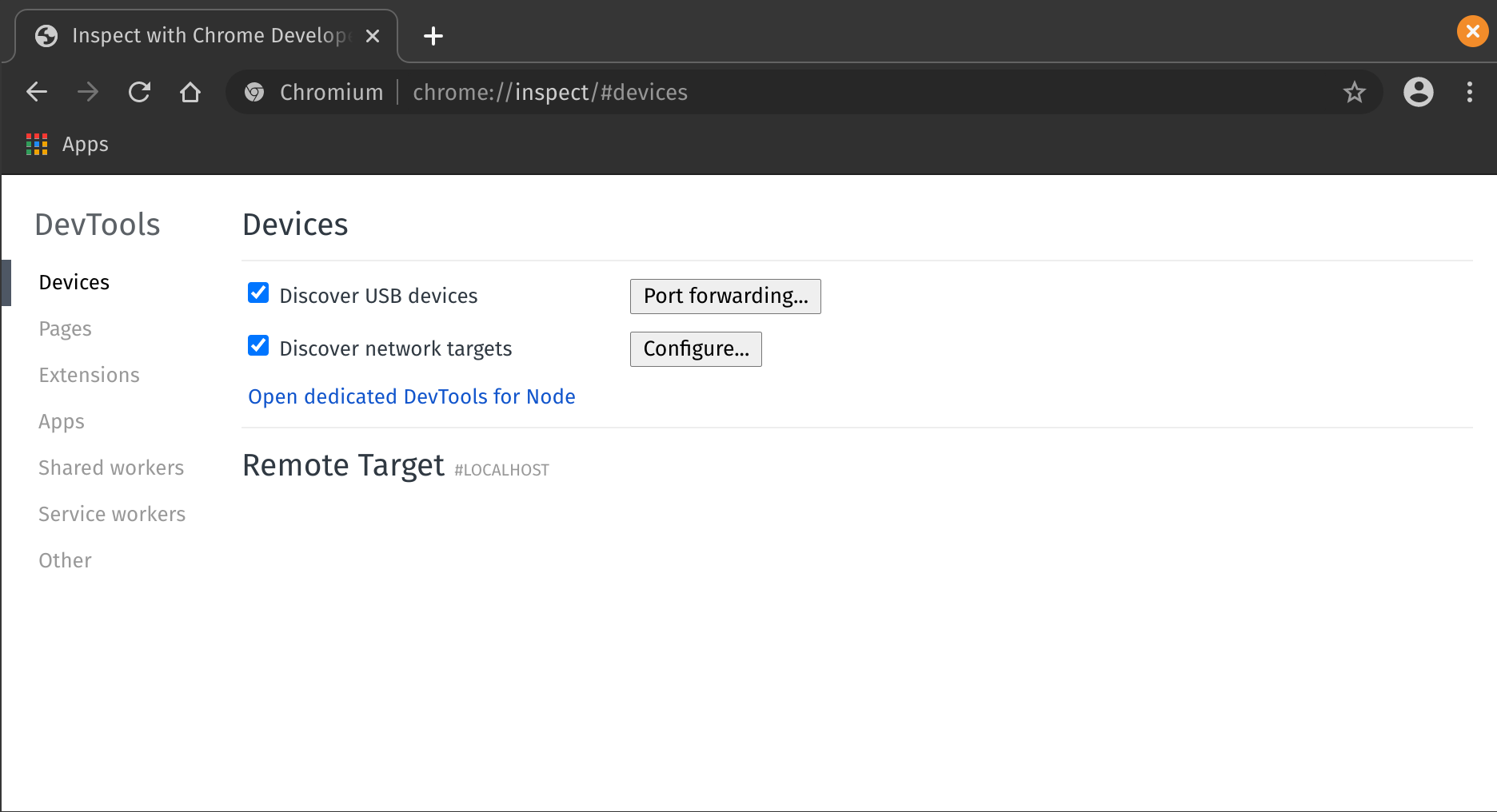A detailed description of the settings menu screen reads:

The image depicts a settings menu, featuring a black bar at the top that houses a circular orange close button on the right with a white 'X' inside it. On the left-hand side of this bar is a tab labeled "Inspect" in white text, followed by "Chrome Develop." Below the black bar, on the left, are several browser-related buttons, including "Chromium" and "Chrome Inspect," along with an eye-catching blue-activated indicator. Immediately below these buttons is a small icon representing apps.

To the right of the black bar's center, a white and black person icon is present. The main section of the window has a white background with predominantly black text. On the left is a list-like panel without a scroll bar; the selected item is “DevTools,” under which other entries like “Devices,” “Pages,” “Extensions,” “Apps,” “Shared Workers,” and “Service Workers” are slightly grayed out.

The central part of the menu is labeled “Devices,” with sub-sections including “Discovery” and “USB Devices.” A blue check mark is present next to the “USB Devices” option, indicating it is enabled. Adjacent to it is a box with the label “Port Foraging.” Below “USB Devices,” another option titled “Discover Network Targets” also has a blue check mark, and beside it is a “Configure” button. A line of blue text underneath reads “Open Dedicated DevTools for Node,” flanked by two thin horizontal gray lines above and below.

Towards the bottom of the panel, black text states “Remove Target,” with tiny, nearly unreadable accompanying text that likely says “Local Host” or possibly “#LocalHost.”